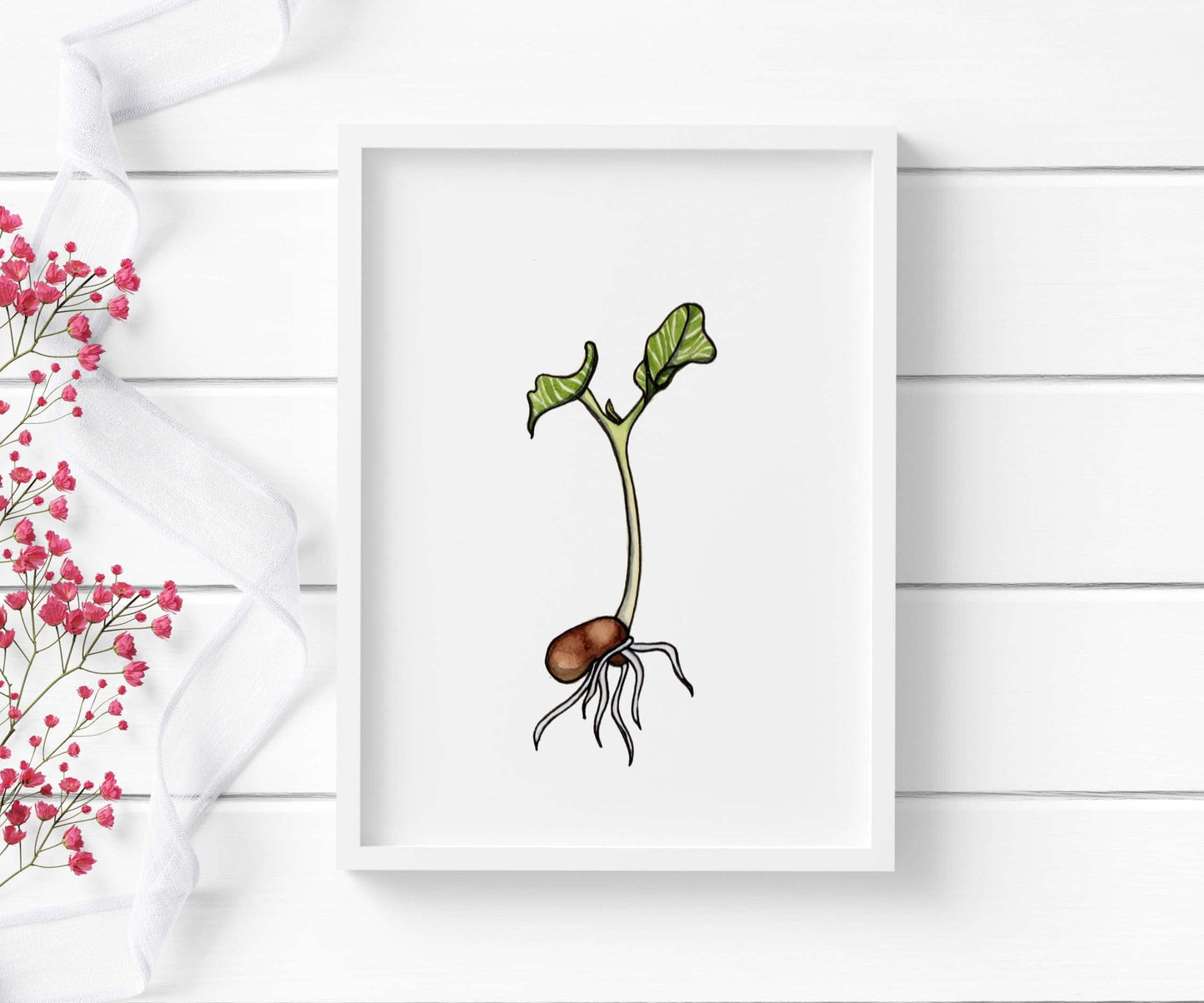The image showcases a white wooden wall with horizontal grooves. Mounted on the wall is a white-framed artwork depicting a detailed ink drawing of a sprouting bean plant. The bean, a rich brown hue, has a light green stem emerging from it, topped with dark green leaves. Light yellow-colored roots extend downwards from the seed. The artwork is set against a stark white background, making the sprouting plant the focal point. On the left side of the image, there is a white ribbon accompanied by a cluster of delicate pink flowers with very thin stems and branches, which occupy about half of the image, adding an elegant contrast to the overall composition.